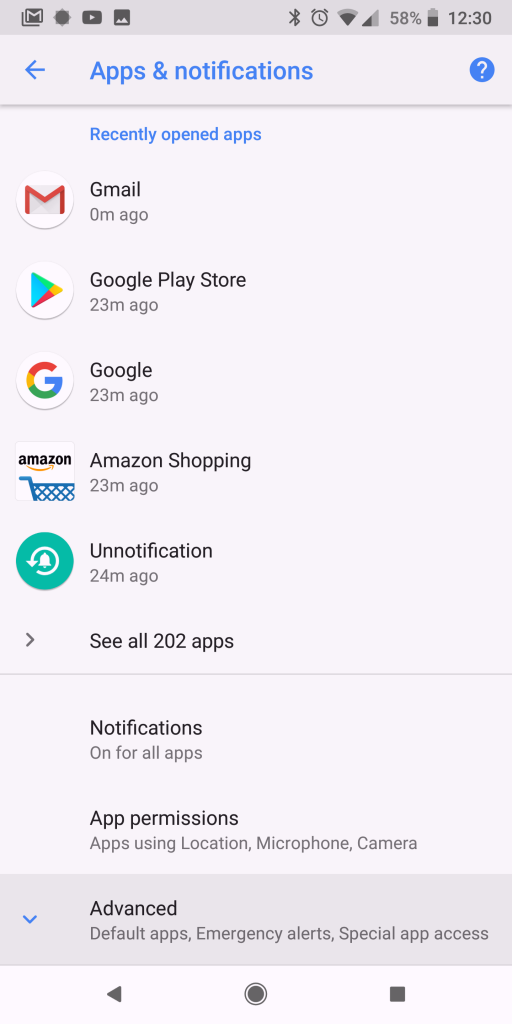The image displays a cell phone screen showcasing the 'Apps & notifications' settings page. At the top, there is a gray status bar that includes icons for Gmail, Sunny, YouTube, Photos, Bluetooth, an alarm clock, Wi-Fi and cellular signal bars, a 58% battery indicator, and the time displayed as 12:30. 

Directly beneath the status bar is a blue header with a left-pointing arrow, the text 'Apps & notifications,' and a circle icon with a question mark inside. Following this is a thin gray line. Underneath, the text 'Recently opened apps' appears in blue, leading to a list of apps aligned to the left. The list includes:
- Gmail, accessed 0 minutes ago
- Google Play, accessed 23 minutes ago
- Google, accessed 23 minutes ago
- Amazon Shopping, accessed 23 minutes ago
- Unnotification, accessed 24 minutes ago

Below the list, the option 'See all 202 apps' is available with a right-pointing arrow next to it.

Separated by another line, the next section mentions:
- 'Notifications on for all apps'
- 'App permissions'
- 'Apps using location, microphone, and camera'

Further down, on a darker gray background, the text 'Advanced' is shown, followed by details such as 'Default apps,' 'Emergency alerts,' and 'Special app access,' with a downward-pointing blue arrow to the left of these options.

At the bottom of the screen, there are navigation buttons that include a left-pointing arrow, a circle, and a square, all displayed in black.